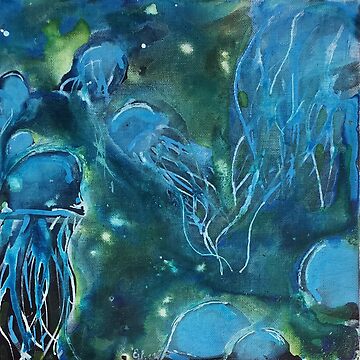The image is an abstract painting depicting numerous jellyfish floating gracefully in water that has a mix of cool, dark shades of grayish-blue and light patches of green. The sun's reflection creates white speckles throughout the water, enhancing the overall ethereal atmosphere. The jellyfish are primarily blue with some white highlights, displaying a reflective, transparent quality. One jellyfish, positioned closer to the viewer in the upper right corner, has more pronounced tentacles, while the rest are scattered across the image. Some jellyfish are fully visible, while others are only partially seen, adding to the mystical and dynamic feel of the artwork.